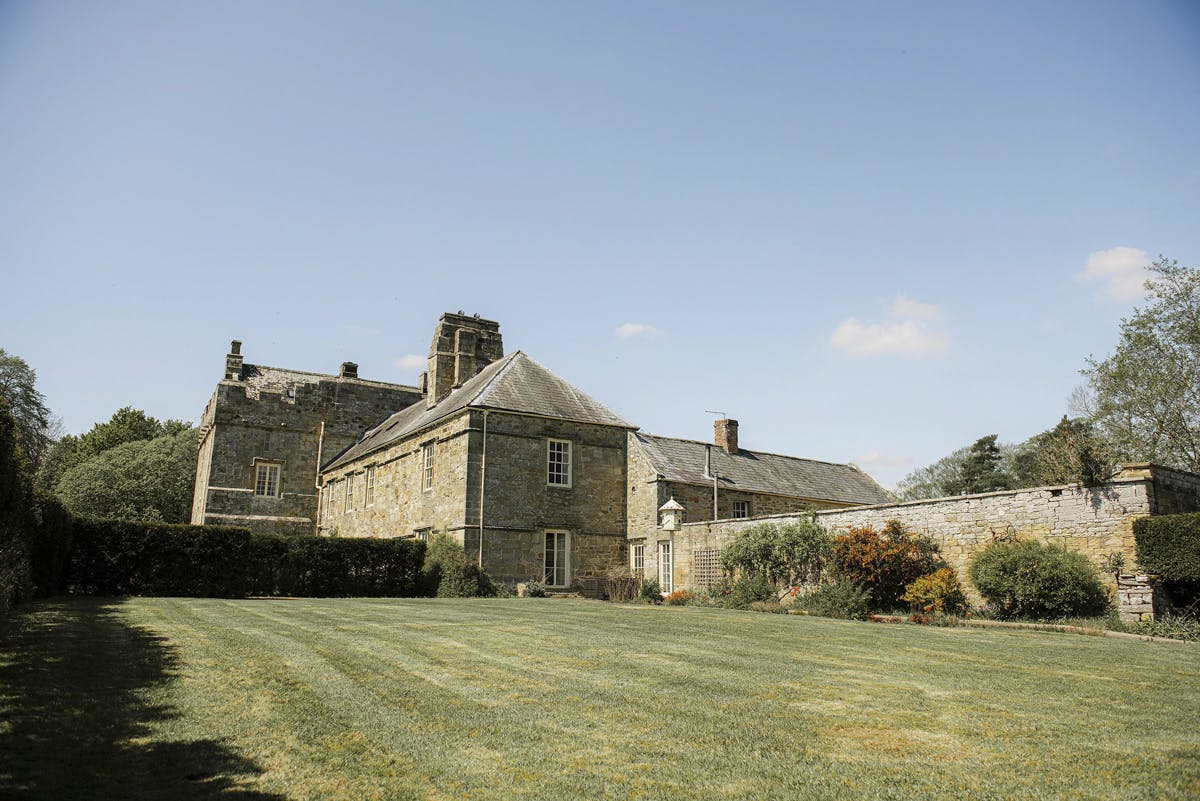The image showcases a stately two-story manor, likely located in rural England, constructed from a blend of brown and gray stone. The building features a gray shingled roof and possesses a rectangular main section with a short oblong wing projecting from the left front, and another smaller wing or possibly a wall extending from the right front. Rows of windows line the upper story, while a meticulously manicured lawn stretches out in front. A hedge partially obscures the lower part of the building on the left side, with additional bushes lining a brick wall on the right, leading to a smaller structure that might be one or two stories high. The scene is set under a clear, sunny blue sky, capturing the timeless essence of this historic, although somewhat faded and weathered, building. In the background, trees frame the scene, enhancing the quaint, rural charm of the landscape.